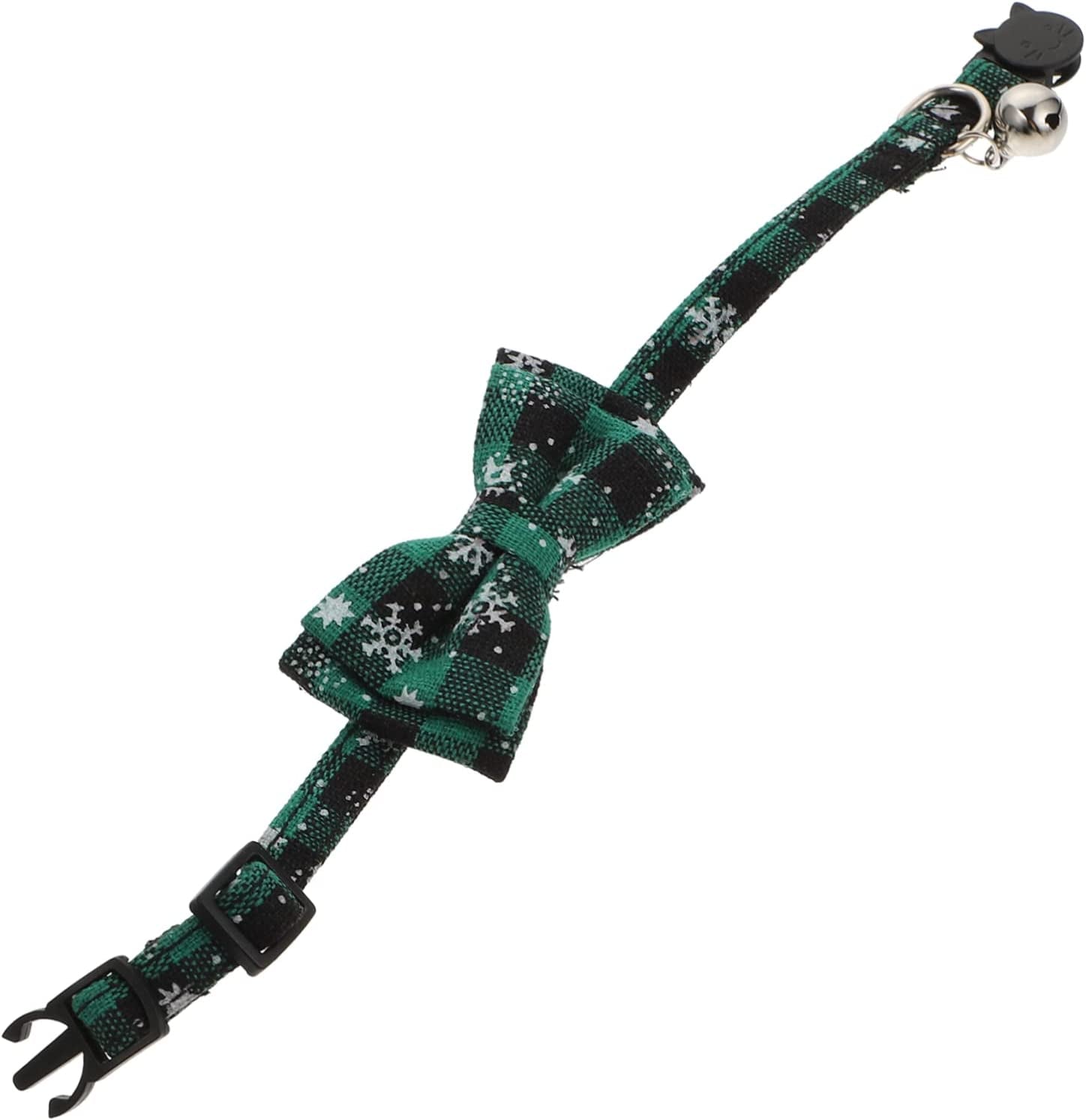A product photograph showcases a festive pet collar, likely designed for a cat. The horizontally aligned image prominently features a plaid green and black patterned fabric with a grainy texture, detailed with white snowflakes, dots, and stars. This fabric forms a bow tie situated diagonally, with the right side slightly elevated. The bow tie's pattern, evenly spread across the cloth, displays two sides of the ribbon in foreground and background, creating symmetrical triangles that taper inward.

On the far left, the collar includes a black plastic three-pronged buckle adjuster for length customization. Adjacent is a three-pronged attacher, convex on both outer sides and straight in the middle, designed to snap securely into a fastening component on the opposite end. Towards the far right, a silver metal bell dangles from a small ring attached by a slender chain. This ring is fastened near a unique cat-head-shaped black plastic clasp, identifiable by its two raised triangular ears.

The absence of a border around the image, combined with its clean white background, draws all attention to the detailed craftsmanship and festive design of the collar. This bow tie-adorned collar integrates both vintage and contemporary styles, making it a charming holiday accessory for any pet.